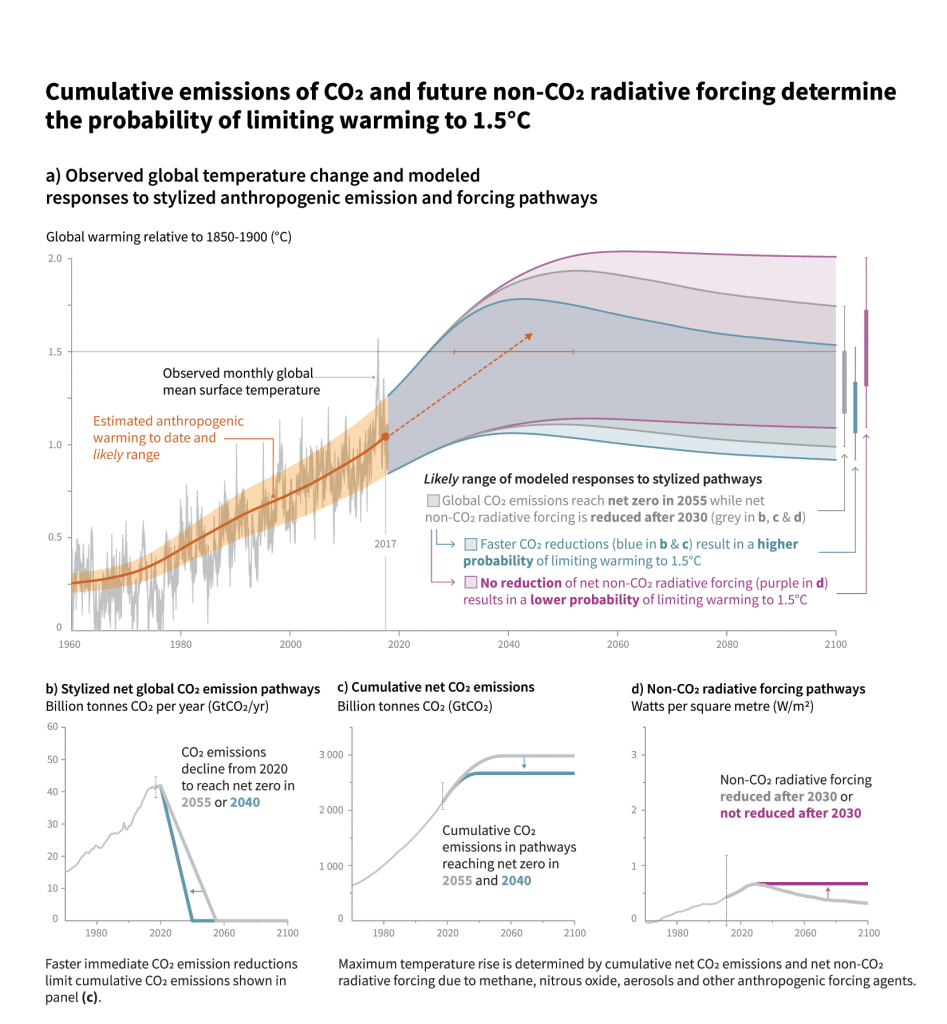Set against a stark white background, the image presents four distinct diagrams and charts that collectively illustrate complex climate data. At the top, a header states: "Cumulative emissions of CO2 and future non-CO2 radiative forcing determine the probability of limiting warming to 1.5 degrees Celsius." 

Below this, a secondary heading reads: 
"A. Observed global temperature change and modeled responses to stylized anthropogenic emission and forcing pathways." 

The first diagram beneath this secondary heading shows the global warming relative to 1850 to 1900 Celsius, charting data from 1960 through projections to the year 2100. The vertical axis measures from 0 to 2.0 degrees Celsius and plots the observed monthly global mean surface temperature alongside a likely range of modeled responses to different stylized pathways.

Directly beneath, three more diagrams detail various climate variables:
- The second diagram illustrates "Stylized net global CO2 emission pathways."
- The third focuses on "Cumulative net CO2 emissions."
- The fourth depicts "Non-CO2 radiative forcing pathways."

Each diagram meticulously portrays pivotal data, contributing to a comprehensive understanding of how cumulative CO2 emissions and non-CO2 radiative forcings influence global warming and the critical probability of limiting it to 1.5 degrees Celsius.